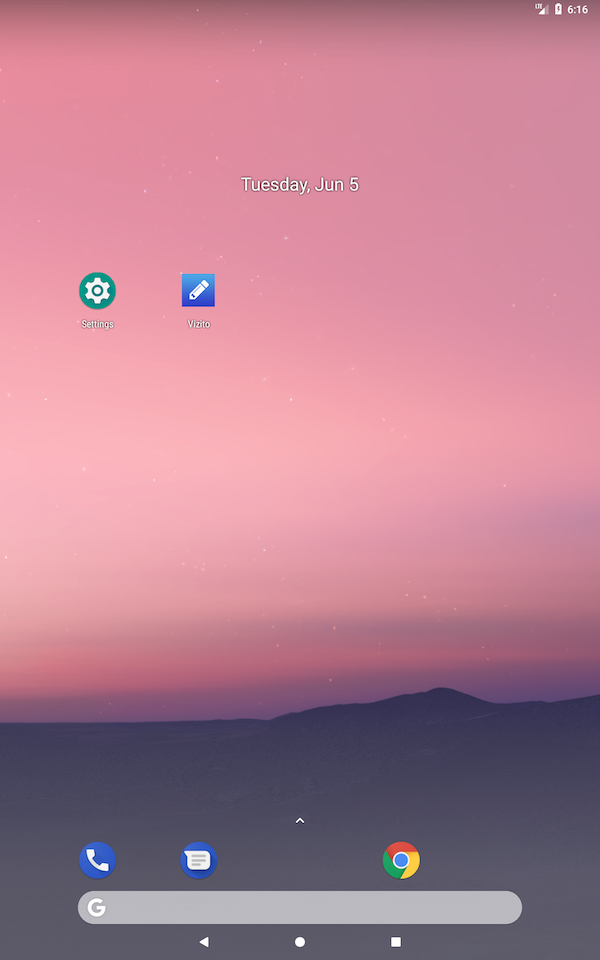This image features the home screen of a cell phone with a visually striking gradient background. At the top, the main color transitions from a pinkish hue to a delicate peach tone as you scroll downward. Further transitioning towards the bottom, the background shifts to a deeper brown shade. In the upper right-hand corner, the screen displays a fully charged battery icon indicating the phone is plugged in, alongside the time, which reads 6:16. 

Centrally positioned, the date is prominently displayed as "Tuesday, June 5th." Below this is a green area designated for settings. Next to it is an application icon featuring a pencil inside a blue square labeled "Vizito." At the bottom of the screen, there are various interactive icons, including a phone, a speech bubble, and what appears to be the Google or possibly Firefox browser icon.

The background as a whole is reminiscent of a tranquil evening sky, blending from a soft pink hue at the top to darker shades at the bottom, complemented by a brown mountain that adds a naturalistic touch to the scene. The overall composition provides a visually pleasing and functional home screen interface.